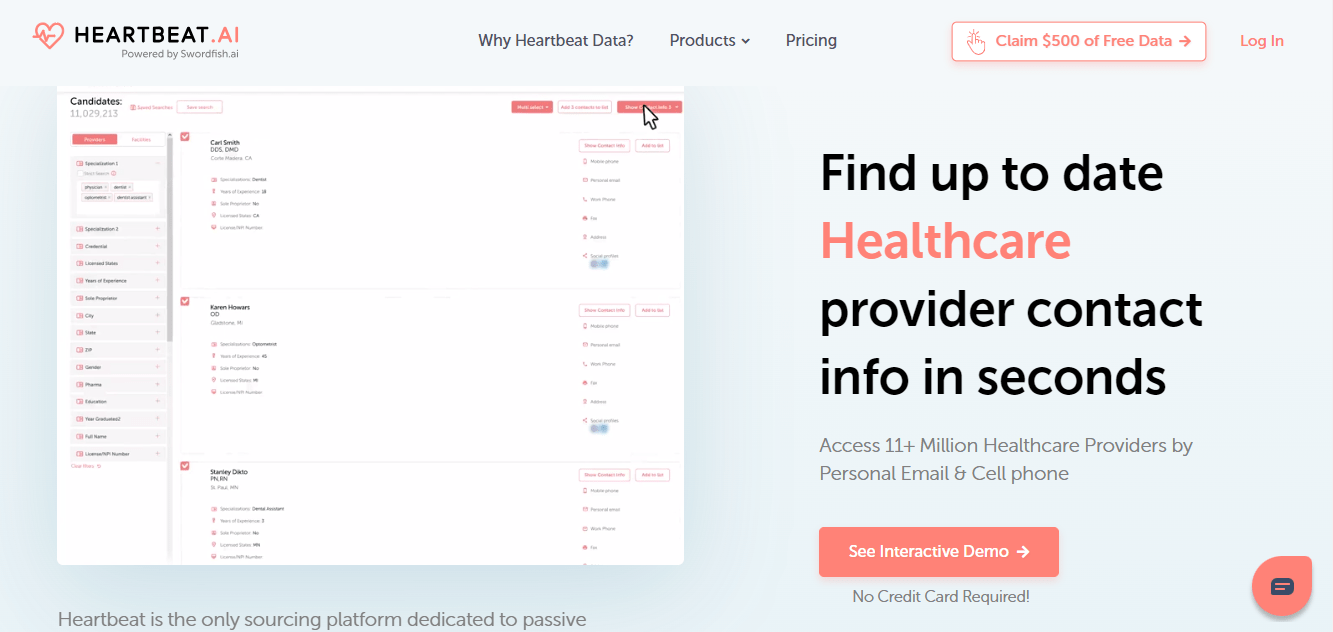The promotional image for Heartbeat.ai features a detailed and visually engaging layout. In the upper left corner, set against a grayish-blue background, a red heart with a lifeline graphic prominently displays. The text "heartbeat.ai powered by swordfish.ai" is positioned next to the graphic. Directly below this, clickable options labeled "Why Heartbeat Data?", "Products", and "Pricing" are neatly presented.

In the upper right corner, a red button invites users to "Claim $500 of Free Data," accompanied by a red "Login" link. Below this offer, the text highlights the platform's capabilities: "Find up-to-date healthcare provider contacts info in seconds. Access 11+ million healthcare providers by personal email and cell phone." A bright red button labeled "See Interactive Demo - No Credit Card Required" is prominently featured.

In the bottom left corner, the image asserts, "Heartbeat is the only sourcing platform dedicated to passive..." with the textual description trailing off. Adjacent to this, a white window showcases a preview of the platform's interface. This section highlights individual candidates like "Carl Smith" and "Karen Hoover" along with several checkboxes for various filter options, demonstrating the user-friendly data filtering capabilities of Heartbeat.ai.